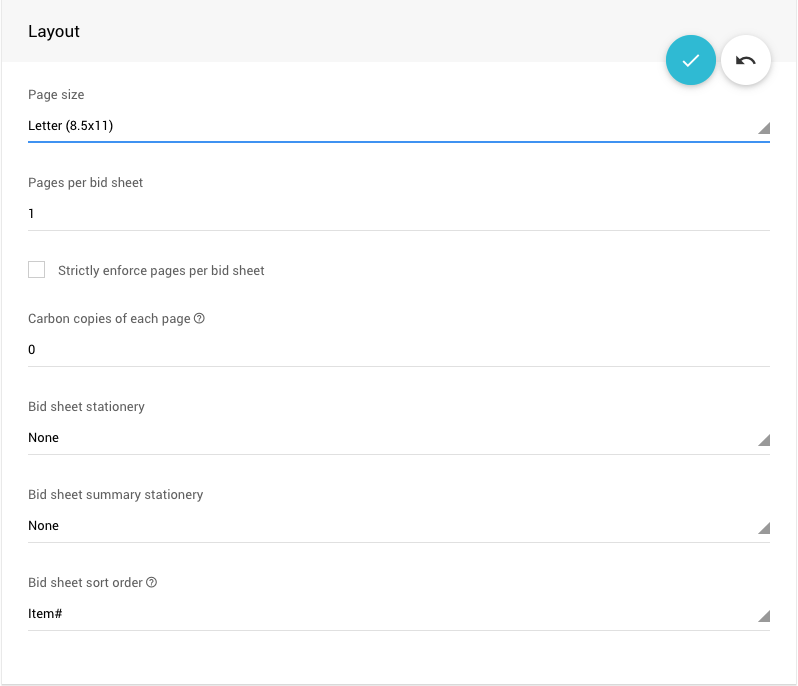This image features a screenshot of a computer interface displaying a layout settings page. The background is predominantly white, with a gray header at the top labeled "Layout." Within this gray header, towards the right, there are two icons: a white check mark inside a circle and a black arrow that resembles a refresh symbol.

Beneath the header, the page is organized into sections separated by thin blue and faint gray lines. The first section specifies the page size as "Letter 8.5 by 11." Moving down, the next section is titled "Pages per Bid Sheet," which indicates a value of "1," with an option for "Strictly enforced pages per bid sheet" left unchecked.

Further down, the setting "Carbon copies of each page" is set to "0." Below this, separated by another faint gray line, the option "Bid Sheet Stationary" is marked as "None." Another faint gray line follows, leading to the next setting, "Bid Sheet Summary Stationary," which is also set to "None."

At the bottom of the page, after another faint gray line, the final section is labeled "Bid Sheet Sort Order," displaying that the sort order is set to "Item Number."